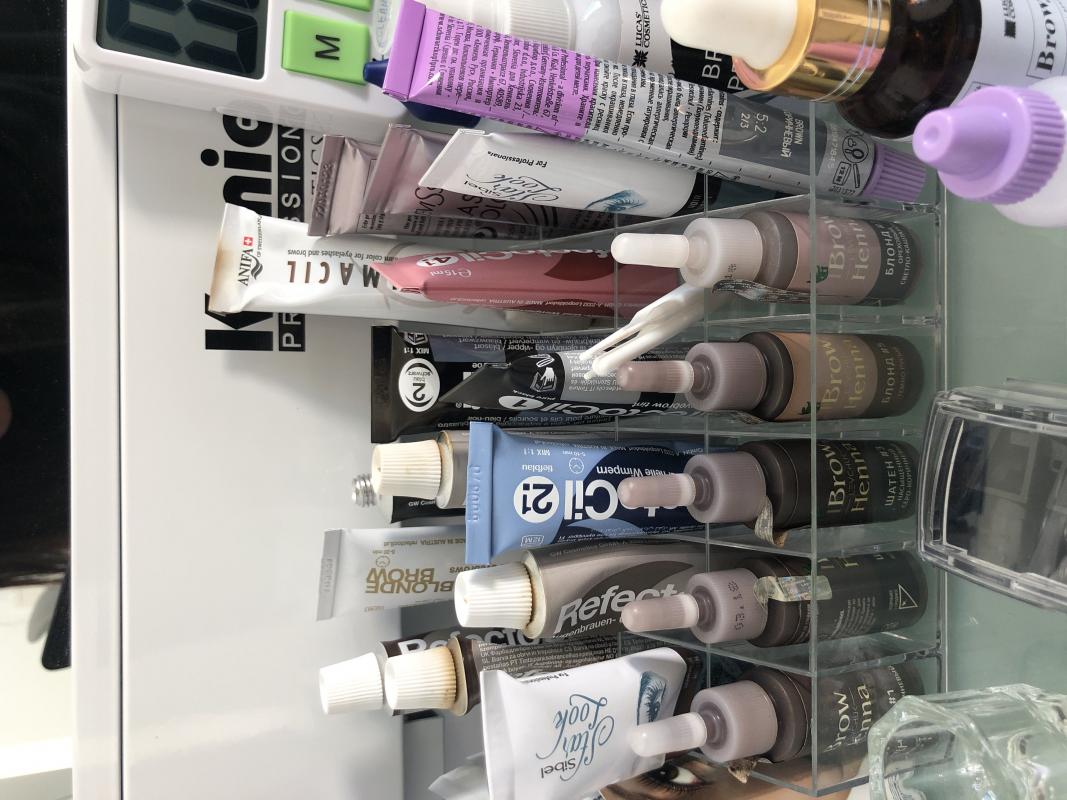The image showcases an organized display of beauty products within a multi-tiered plastic container, positioned atop a glass shelf. Noteworthy is the image’s tilted orientation, with the bottom appearing on the right and the top on the left. The plastic container features several levels, each housing different items.

On the bottom tier, there are five distinct bottles of brow henna ink, each nestled in its own individual compartment. The next level up contains tubes of various other products, also divided into separate sections within the container. 

In the foreground, there is another smaller plastic container with a black accent and a shot glass-like item on its left side. Surrounding the edge of this main container, particularly to the right, are several other miscellaneous bottles. Additionally, a calculator is visible on the far right side, blending into the background and completing the setup.